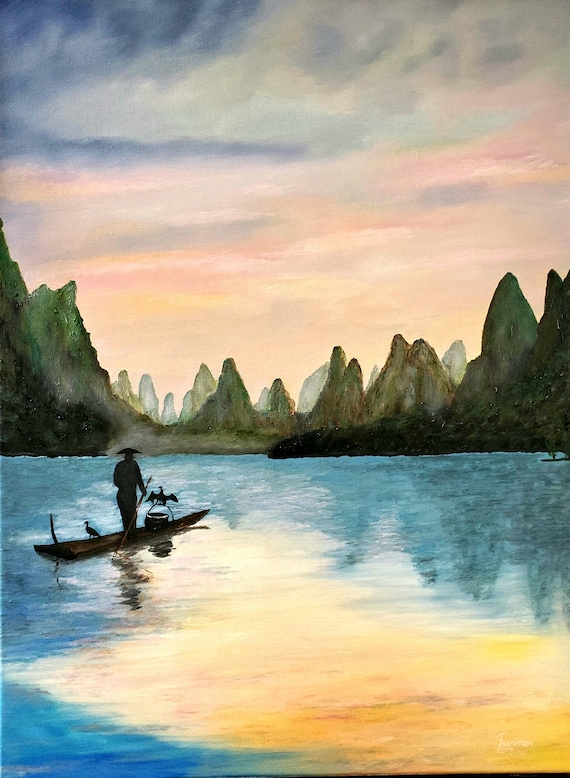The image is a watercolor painting depicting a serene and picturesque scene set on a lake, likely in China. At the center of the image stands a traditional Chinese fisherman on a shallow, flat-bottom gondola. He is poised with a long pole, maneuvering the boat forward. Accompanying him are two cormorants: one with its wings majestically spread and the other perched calmly beside him. This scene illustrates an ancient fishing technique where cormorants were used to catch fish.

The lake's surface mirrors the landscape and sky, creating a tranquil reflection. The background is adorned with lush, mountainous foliage that fades into the distance. Above, the sky is an enchanting blend of pinks, blues, yellows, and subtle clouds, suggesting the time is either twilight or dawn. The soft light of the setting or rising sun casts a gentle glow, tinting the scene in muted yet vibrant hues. This combination of elements—nature, tradition, and time of day—imbues the painting with a sense of peace and timeless beauty.